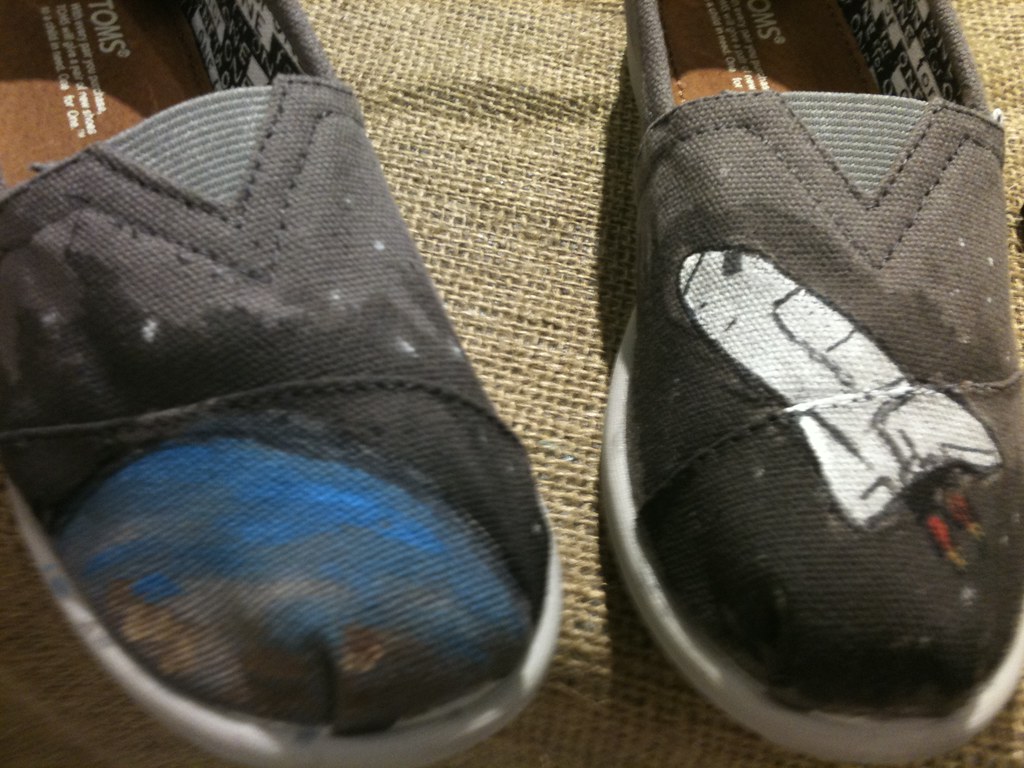This close-up, almost artistic image captures a pair of well-worn Tom's slippers placed on a brown burlap fabric. The slippers, which resemble basic tennis shoes, are predominantly dark gray with white soles and brown interiors. The left slipper, oriented on the right side of the image, features an abstract painting of Earth with a background of space depicted in dark gray with white speckles representing stars. The right slipper, positioned on the left side, showcases a white space shuttle with flames streaming from its back, also set against a star-speckled dark gray background. The intricate patterns and the well-loved appearance of the slippers add a captivating, rustic charm to the photo.